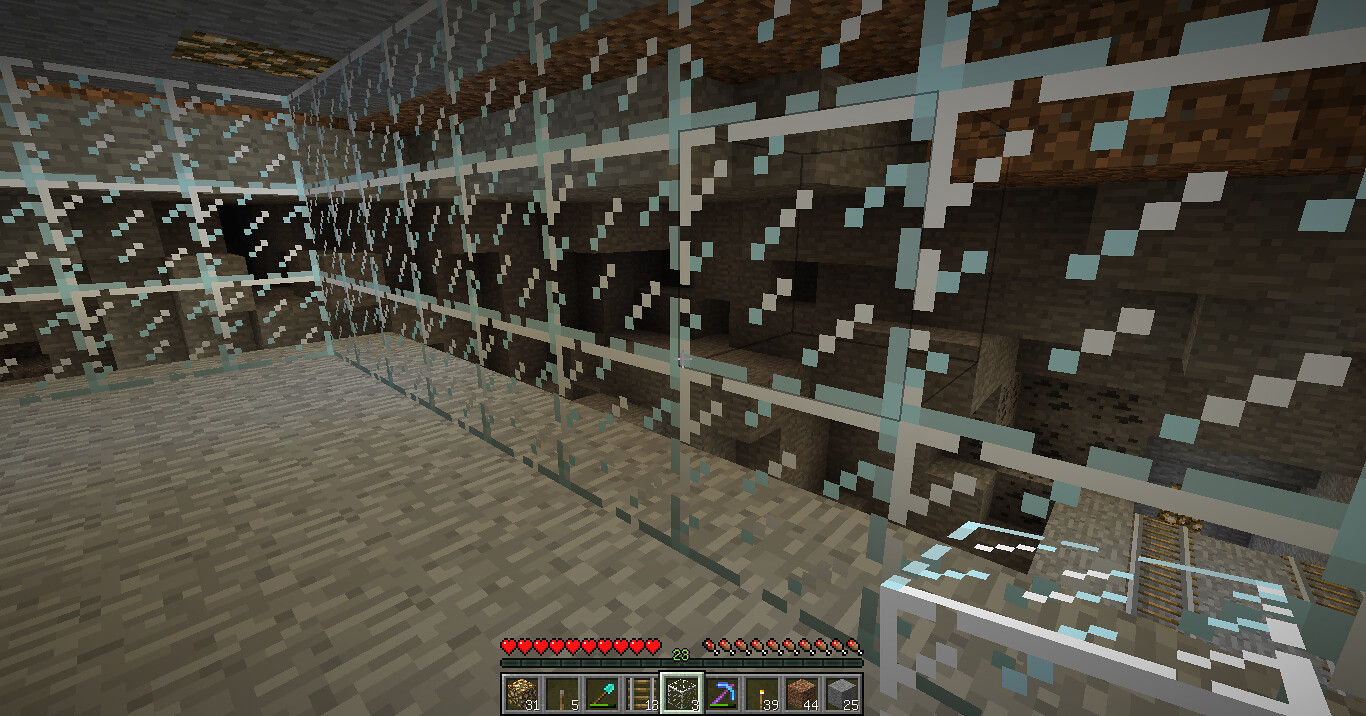The image is a still from a video game displayed in a rectangular format. The graphics are rudimentary, featuring pixelated art. The scene lacks characters and instead displays a pixelated environment with a light brown floor. At the bottom of the image, there is a small menu or HUD (Heads-Up Display) area. This section includes several hearts, potentially indicating health points, along with various icons that may represent food items or other resources. These icons likely signify health, energy, or similar metrics, though their exact purposes are unclear. Below the hearts and icons, there are squares each containing a symbol accompanied by a number, but the specific meanings of these symbols and numbers are not discernible from the image.